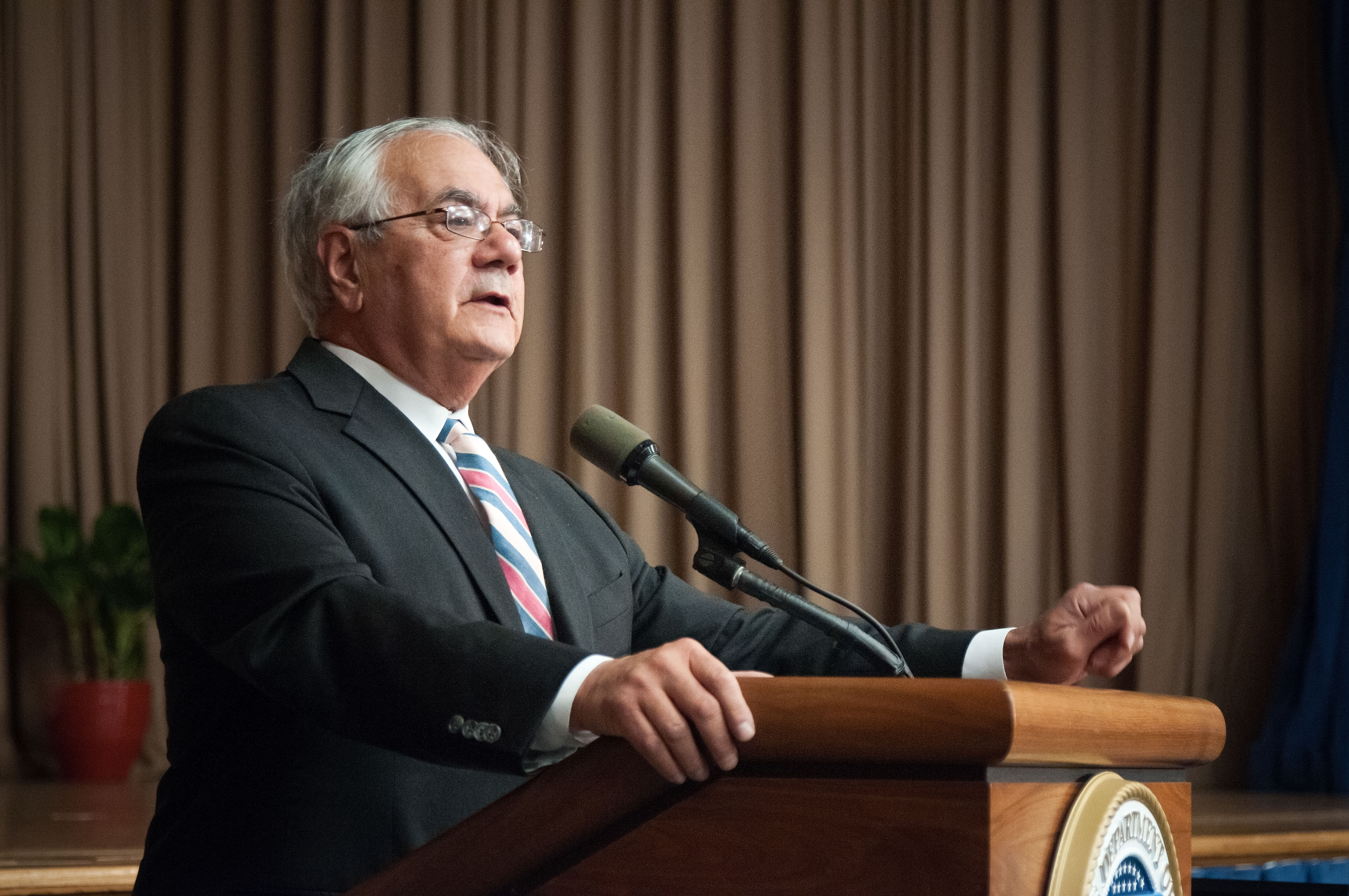The image depicts Barney Frank standing behind a brown podium, delivering a speech at what appears to be a conference or convention. He is dressed in a dark suit jacket with a white collared shirt and a tie striped with blue, red, and white. His gray hair and wire-rimmed glasses complement his appearance, suggesting he is in his 50s or early 60s. Barney Frank is captured mid-speech, with his left hand slightly above the podium and his right hand resting on its side. A blue emblem with an indistinguishable white inscription adorns the front of the podium. Behind him, a large brown curtain forms the backdrop, draping down to the stage. Under his right shoulder, a potted plant with green stems and leaves in a red pot adds a touch of color to the scene. The overall setting indicates a formal event.